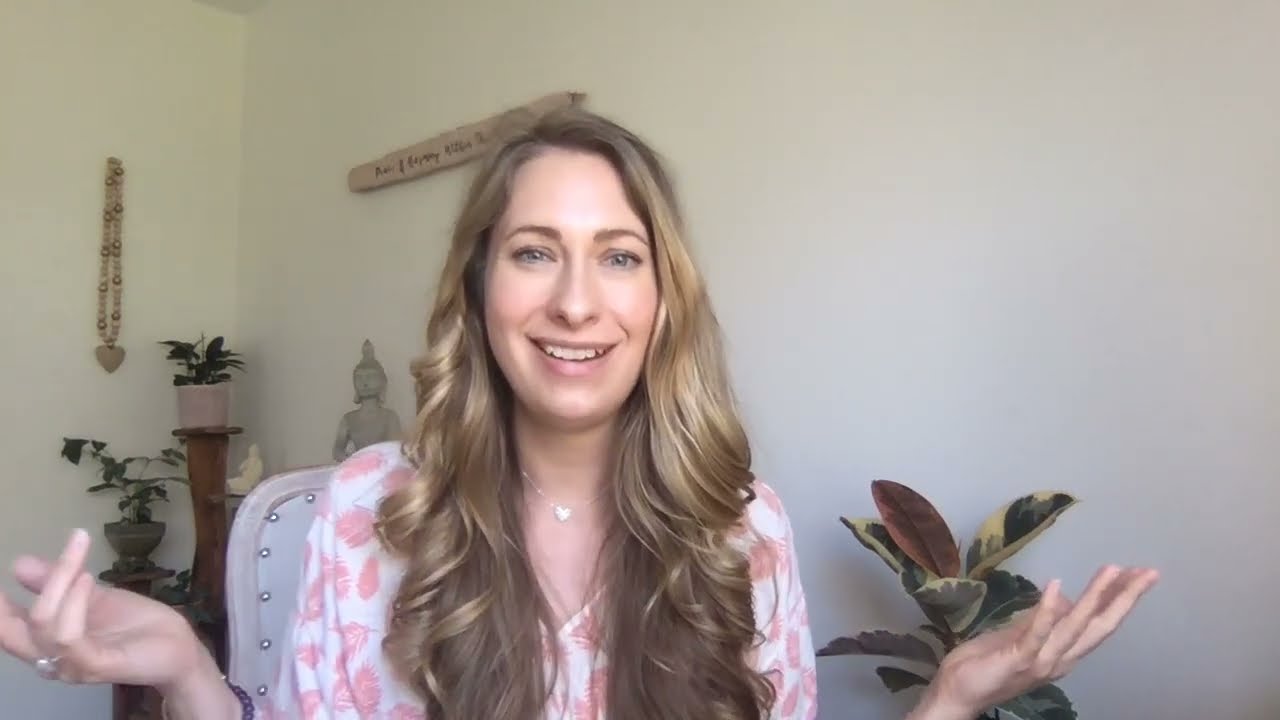In the image, a woman with long, sandy brown hair parted to the side and blue eyes is seated in a white chair adorned with silver studs. She is smiling gently at the camera, her hands raised to her sides with palms facing up, as if in a questioning or contemplative gesture. She wears a white V-neck shirt decorated with pink leaf patterns, and a silver dainty necklace with a small heart pendant rests around her neck.

The setting appears to be indoors, likely in a living room or bedroom, with natural light suggesting it's daytime. The background features a beige wall adorned with a large, wooden beaded necklace and a brown sign with illegible text. A distinctive plant stands to her right, characterized by large green leaves with yellow and red hues, while to her left, there is another plant set on a tiered wooden stand. Behind her, a gray stone Buddha statue adds a serene element to the scene. The overall color palette of the image includes tans, light browns, peach, pink, white, green, and brown, creating a warm and inviting atmosphere.